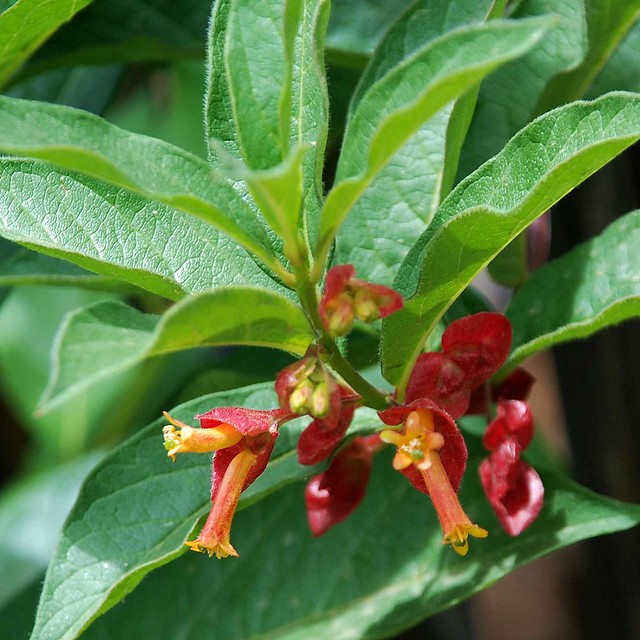This close-up photograph captures the Twinberry honeysuckle in stunning detail. The image showcases a cluster of narrow, pointed, and slightly cupped green leaves, each with clearly visible veins and indentations, presented in a brilliant, non-shiny flat green. The leaves dominate the sharpest focus of the photograph, emphasizing their texture and the intricacies of their structure. Amid this verdant display, the honeysuckle flowers emerge, freshly opened, with vibrant red and orange hues. The flowers, slightly out of focus, protrude from the green buds, showcasing yellow stems and small clamshell-shaped structures. The background remains blurred, highlighting the central plant while suggesting a lush, green environment with varying shades of light and dark leaves. The composition draws the viewer's eye toward the striking contrast between the vivid greenery and the rich colors of the honeysuckle flowers.